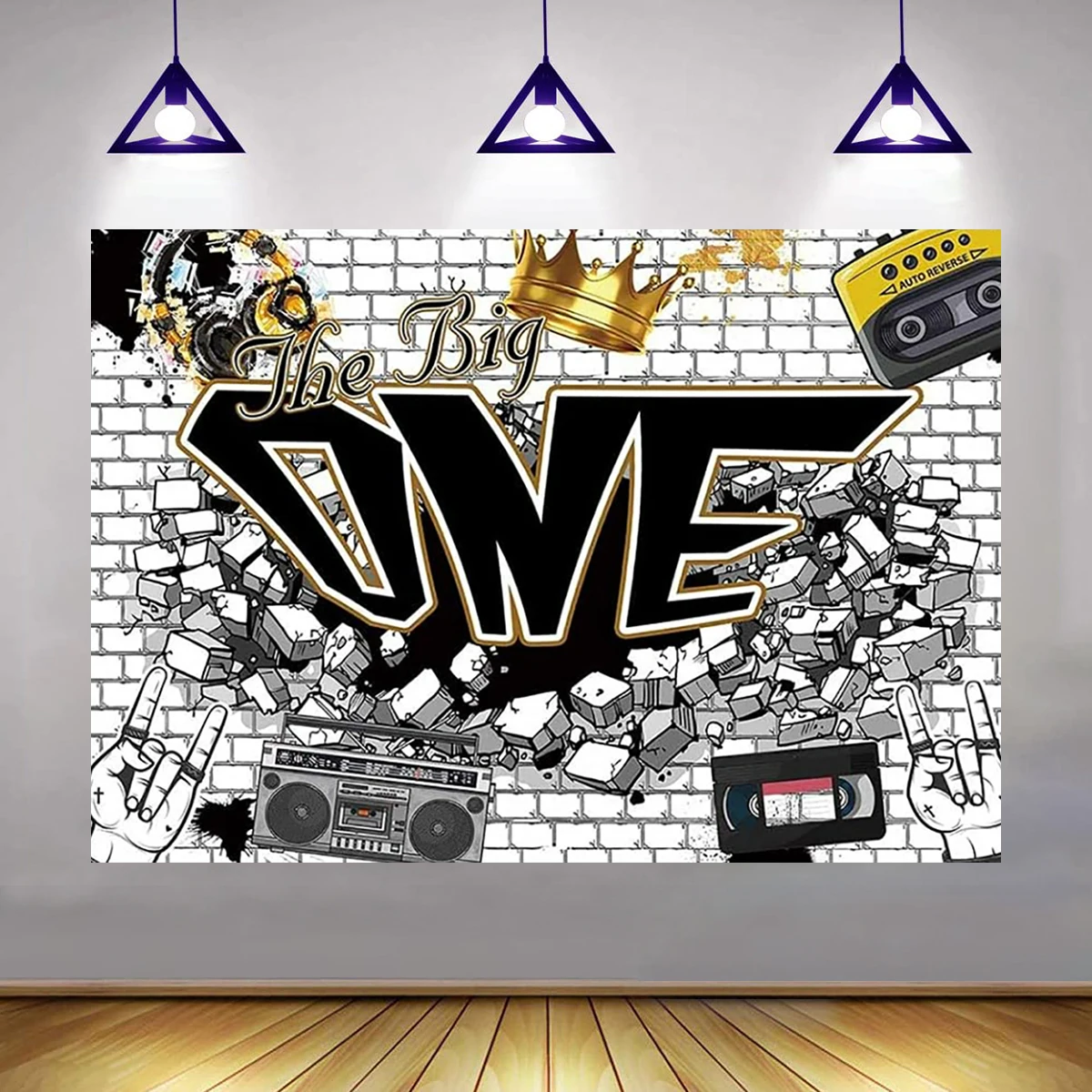The image depicts a stylized, digitally-generated mural set against an interior, light gray wall, covering most of the wall space. Above it, three ceiling lights with black cables and blue triangular fixtures illuminate the mural. The floor beneath is hardwood, running vertically from the viewer's perspective. 

The mural itself simulates a white and gray brick wall with a dramatic, black gaping hole at its center, as if the wall has been forcibly broken. This effect is enhanced by bricks seeming to fly outward from the point of impact. Bold graffiti sprawled across the bricks reads "The Big One," with "The Big" in cursive script and smaller font, and "One" prominently large, outlined in white with a black interior. 

Overlaying this central design are various retro objects: a golden crown sits atop the word "Big" in the center, exuding a regal air; a cassette tape in the upper right corner labeled "Auto Reverse," with a yellow top and gray or black bottom; a black Walkman partially visible; a pair of black, yellow, and red headphones with graffiti-style art in the upper left corner; a portable stereo or boom box with gray, black, and red detailing in the lower left corner; and a black VHS cassette with a gray tape and red label in the lower right. Additionally, disembodied hands in the bottom corners display a "rock on" gesture, adding to the mural's edgy, urban aesthetic.